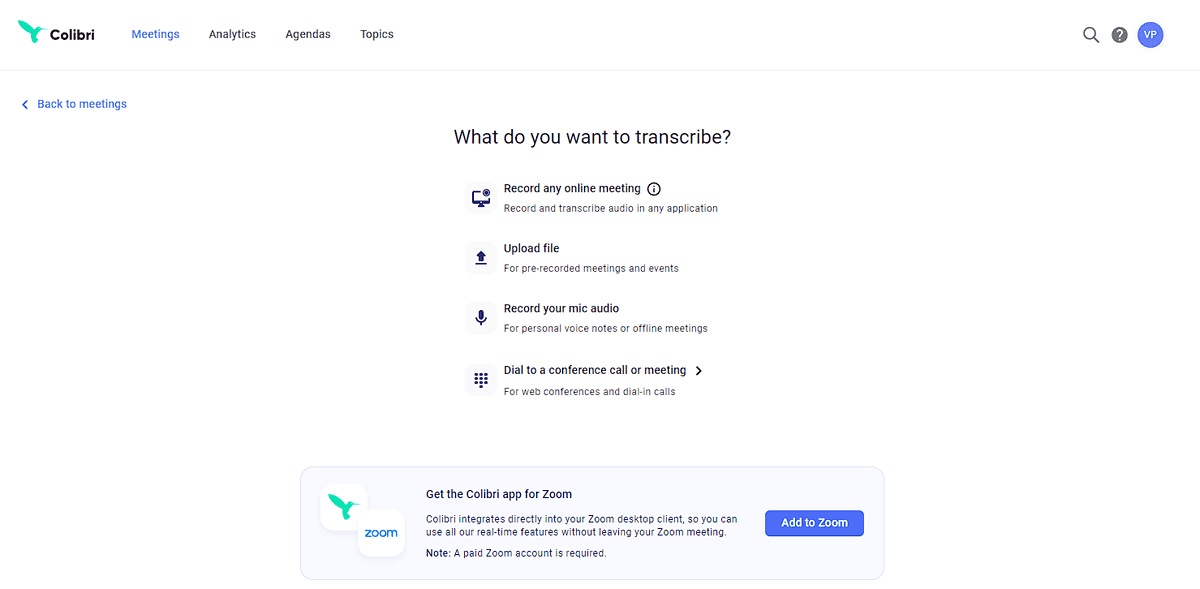In the image, the background is a clean white, providing a stark contrast to the vivid elements dispersed throughout. At the top, there is an illustration of a green bird, which, judging by the context, appears to be a Colibri (hummingbird) although the exact species of bird is unidentified by the observer. Adjacent to the bird is the text "COLIBRI" in bold black letters.

Below this header, there is a series of tabs, the first of which is a blue tab labeled "Meetings", indicating the current section. Other visible tabs, labeled in black, include "Analytics", "Agendas", and "Topics". Towards the top right corner, there is a search bar accompanied by a magnifying glass icon, followed by a gray circle with a question mark, and a blue circle with white text that reads "Repeat".

A subtle gray line runs across the interface, delineating sections. On the left side, a blue arrow accompanied by the text "Back to Meetings" directs users back to the main meetings page. Below this, in black text, a series of options and descriptions are listed under the heading "What do you want to transcribe?" It provides various functionalities including recording and transcribing online meetings, recording audio from various applications, uploading files for pre-recorded meetings and events, and recording personal voice notes for offline meetings.

Further down, another section in off-white background elaborates on additional features: dialing into conference calls or meetings for web conferences and dial-in calls. At the bottom of this section, the green bird logo appears again next to the text "Zoom". It promotes the Colibri app for Zoom, explaining its direct integration with the Zoom desktop client. The final note clarifies that a paid Zoom account is required to access these features.